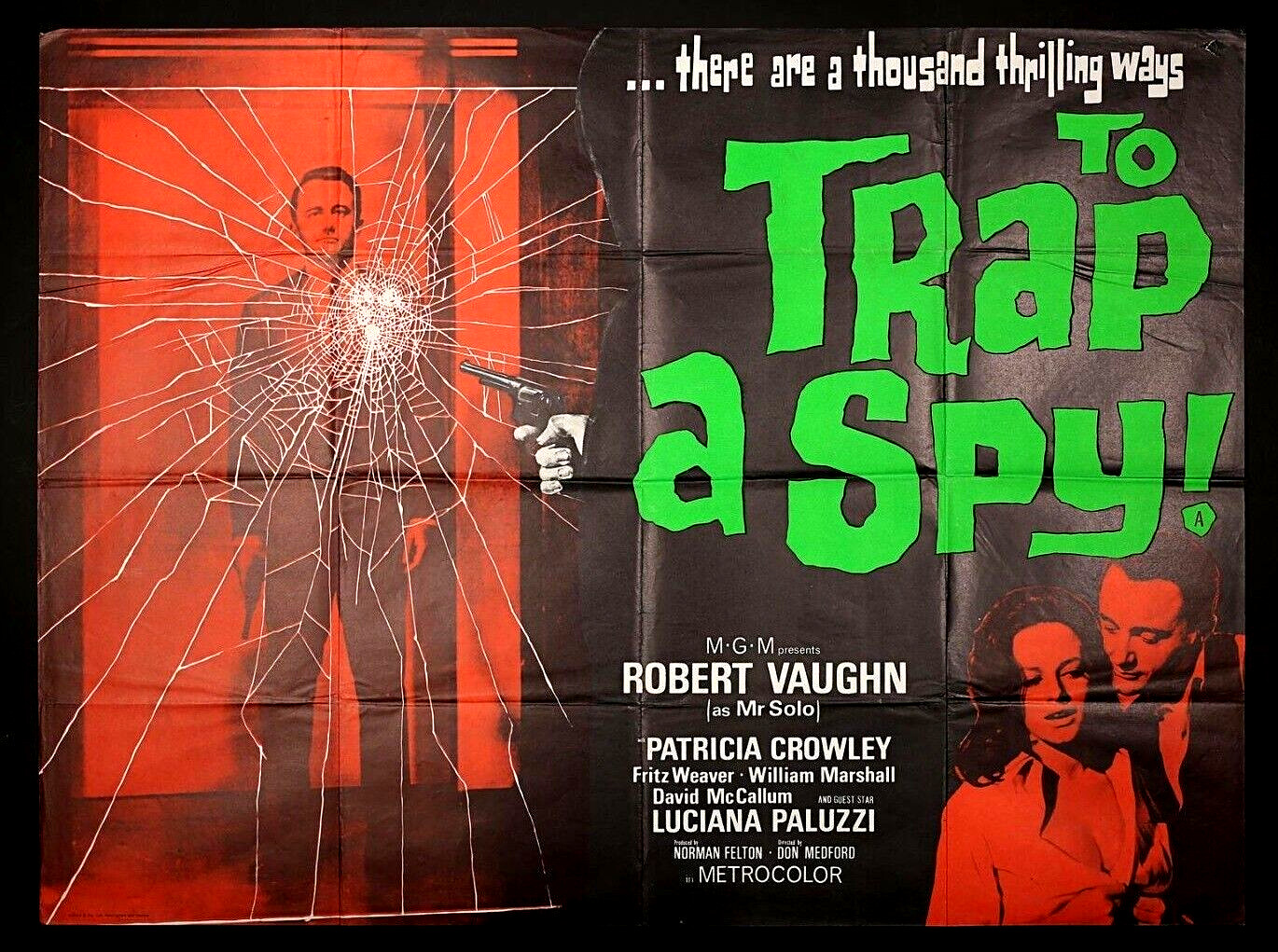This horizontal rectangular movie poster, likely from the 1960s or 1970s, features bold colors and dramatic imagery consistent with spy thriller aesthetics. The overall background is dark, predominantly black or dark gray, with red, green, and white as the main colors used for emphasis and text. 

On the left side of the poster, there is a striking image of a man standing behind a shattered glass panel, holding a gun in his right hand. The glass appears to have been shattered by a bullet, emphasizing the dramatic tension of the scene. Behind him, red light spills through, adding to the heightened sense of danger. This man, identified as Robert Vaughn, plays Mr. Solo, a central character in the movie. 

Above this intense scene, bold text in white and green reads: "There are a thousand thrilling ways to trap a spy!" This tagline sets the tone for the viewer's expectations. 

The lower right corner of the poster features another image, this time of Robert Vaughn alongside Patricia Crowley, both illustrated with a red cast against their figures. This adds a sense of continuity and thematic cohesion to the overall design.

Centered at the bottom of the poster, white text announces the primary cast: "MGM presents Robert Vaughn as Mr. Solo, Patricia Crowley, Fritz Weaver, William Marshall, David McCallum, and Luciano Paluzzi." Names of other contributors, such as Norman Felton and Don Medford, are also present, highlighting their involvement. The entire image is noted to be in 'MetroColor,' suggesting a vibrant, colorful presentation typical of the period.

Overall, the poster is a compelling mix of visual storytelling and promotional text, emphasizing high-stakes espionage and star power.